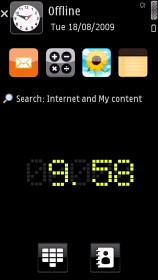This detailed screenshot captures a mobile phone interface with a primarily black wallpaper. At the top of the screen, there is a small white X in the top left corner, followed by a clock icon to its right. Centered at the top is the word "Offline," and next to it, "Tuesday 18-08-2009" displays the date.

Below this header, four icons are arranged horizontally: an orange mail icon, a calculator icon featuring plus, minus, multiplication, and division symbols, a photos icon represented by a sunflower against a blue sky, and a notepad icon. 

Under these icons is a search bar with a magnifying glass icon labeled "Search Internet and My Content." 

Towards the bottom, the current time, displayed in a neon green, pixelated font reads "9.58," unusually separated by a period instead of a colon.

At the very bottom of the screen, two more icons are present: one resembling a black and white grid, likely representing a keypad, and another depicting a notebook with a person silhouette, likely indicating a contact list or address book.